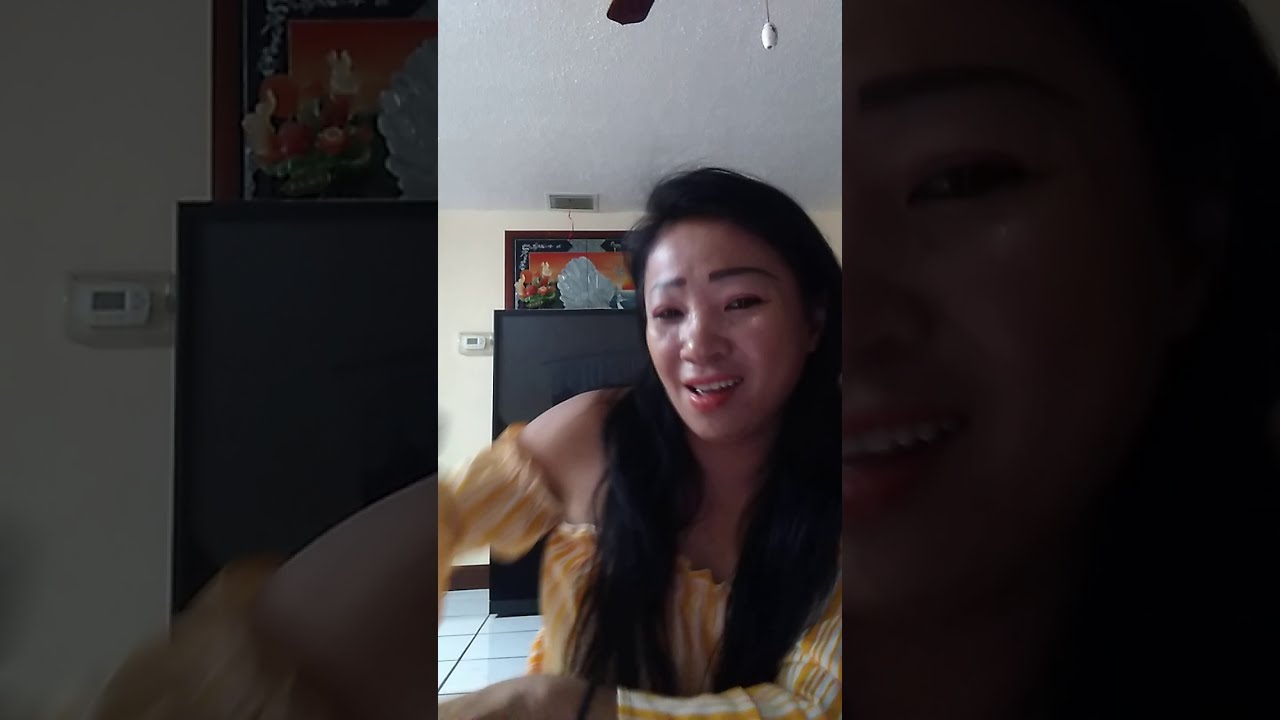In this image, we see an Asian woman, possibly in her late 30s or 40s, with very long black hair cascading down to her chest. She is seated slightly leaning to one side and appears to be making a complex facial expression that could be interpreted as a frown or a tentative smile, with her mouth open just enough to show some emotion. She is wearing a blouse that exposes her shoulders but has sleeves, characterized by its off-the-shoulder design and light yellow color with darker vertical stripes. Her hair falls gracefully over her shoulders in the front.

The background details hint that she is indoors, possibly in a home or hotel room. The space is quite dim and the photo is noticeably blurry and unfocused, making it hard to discern all the details clearly. The floor beneath her features white tiles with black grout, and the ceiling is also white with a visible ceiling fan. There is a hint of a television and some wall decor, possibly art or pictures. Additional background details include a thermostat and parts of a shelf with items on top, reinforcing the sense of an indoor residential or accommodation setting.